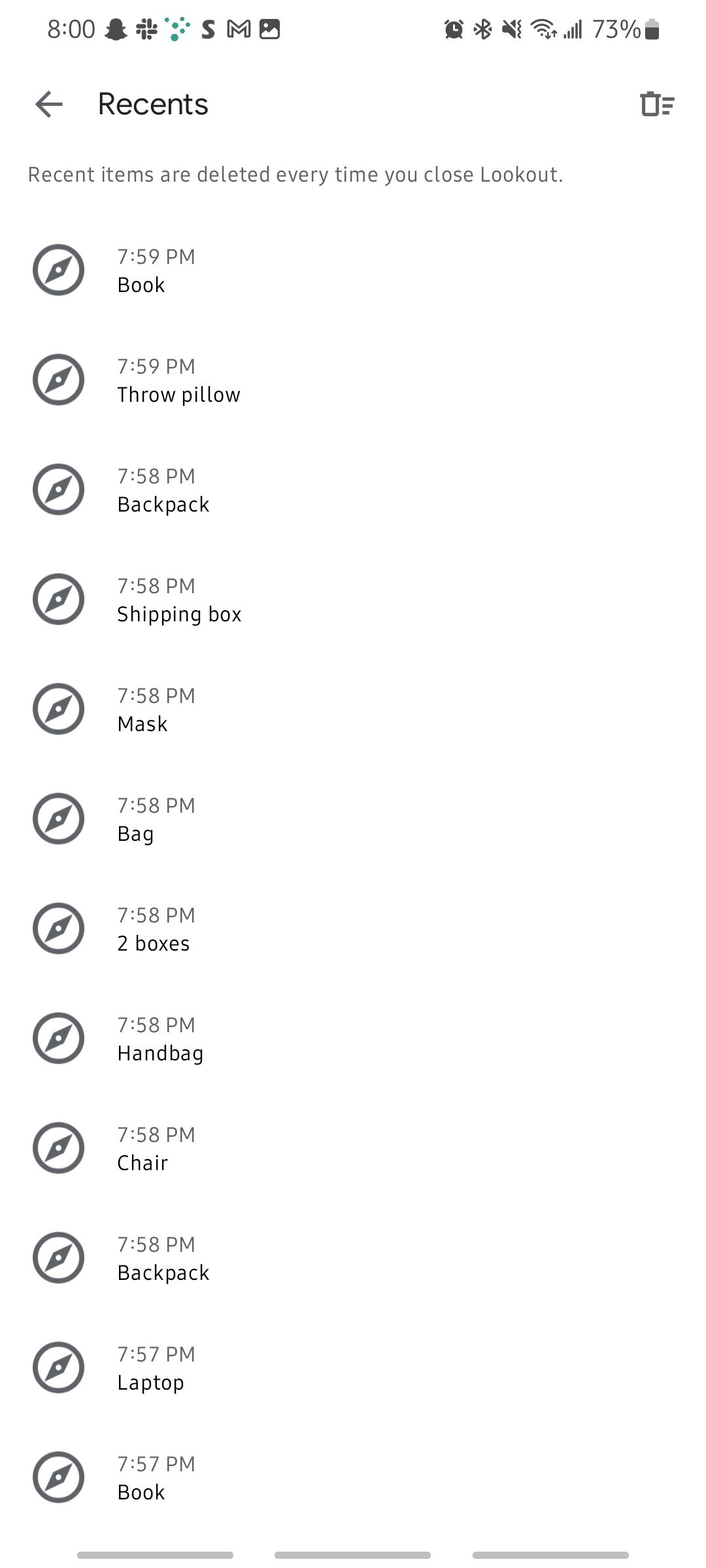Screenshot of the Lookout app displayed on a mobile device. The top-left corner of the screen shows the time as 8:00 PM alongside several status icons, including the Snapchat ghost and the Gmail icon. On the right side of the status bar, the battery indicator reads 73%. The main part of the screen shows the Lookout app interface with a heading labeled "Recent," and a note that recent items are deleted every time the app is closed. Below the heading is a bulleted list of identified items, each marked with a small black compass icon to the left. The list records times and item descriptions, predominantly household furnishings, as follows: 

- 7:59 PM - Book
- 7:59 PM - Throw pillow
- 7:58 PM - Backpack
- 7:58 PM - Shipping box
- 7:58 PM - Mask
- 7:58 PM - Bag
- 7:58 PM - Two boxes
- 7:58 PM - Handbag
- 7:58 PM - Chair
- 7:58 PM - Backpack
- 7:57 PM - Laptop
- 7:57 PM - Book

The Lookout app seems to be used for logging and identifying nearby items, presumably leveraging the device's camera and recognition capabilities.